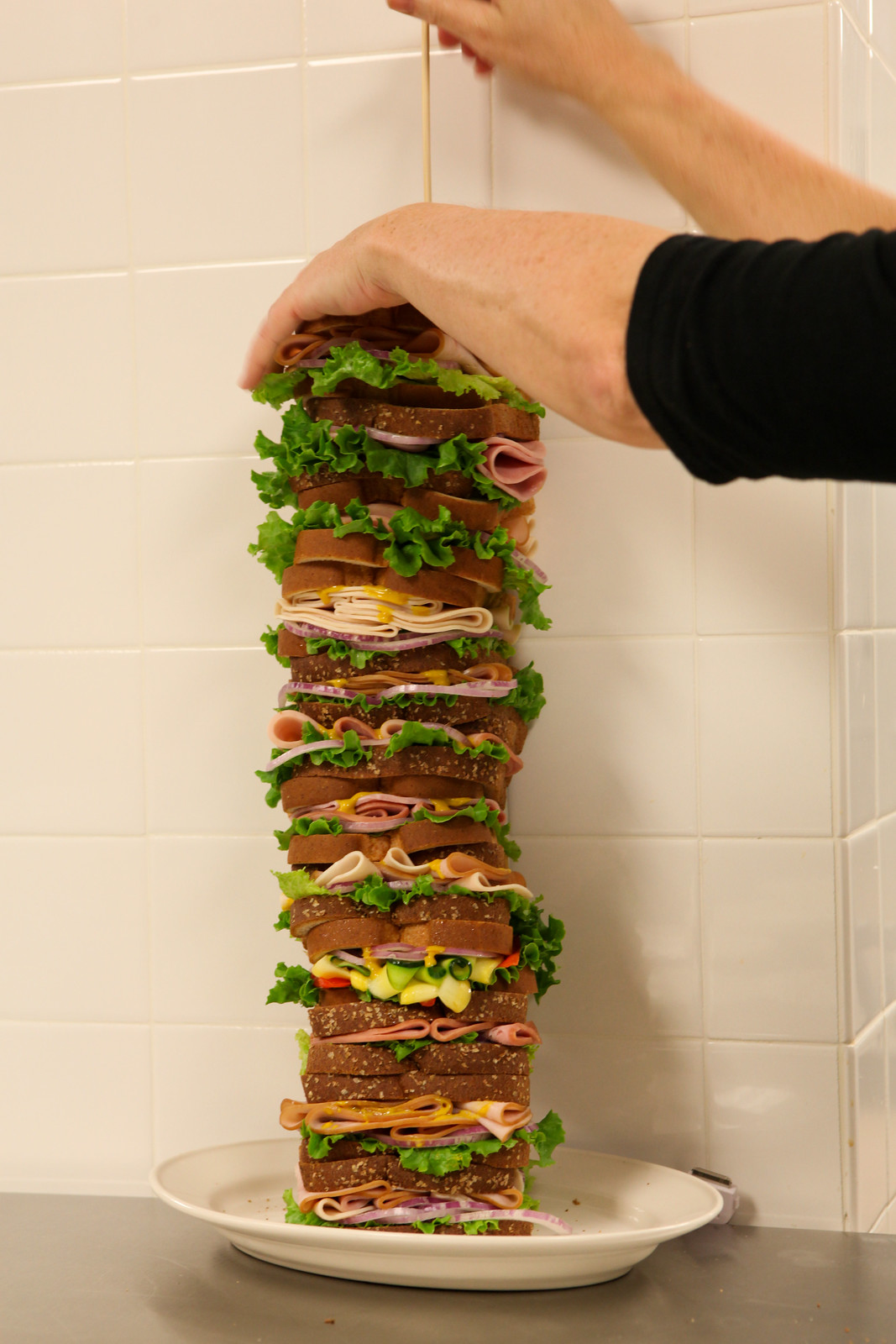In this vibrant color photograph, we see what appears to be a colossal, novelty sandwich, cleverly assembled perhaps for a challenge or simply for fun. The setting, with its white tiled wall in the background, suggests an interior space, possibly a restaurant or someone's home kitchen. The sandwich itself is towering, likely standing about two to three feet high on a white plate placed upon a light brown table.

The sandwich consists of approximately 20 slices of white bread, layered meticulously with a variety of ingredients including bologna, turkey, and slices of ham. Other layers feature cheese, lettuce, and hints of mustard, with some sections also displaying slices of tomato or cucumber. This mega sandwich is capped with the left hand of a person, whose right hand hovers just below, implying they are in the process of stabilizing or presenting it. The person, clad in a long black sleeve, appears to be of Caucasian, European descent, with one hand possibly propped against the wall for balance. The sandwich, an impressive stack reminiscent of a classic Dagwood, showcases an eye-catching array of colors and textures, epitomizing both haphazard charm and structural marvel.